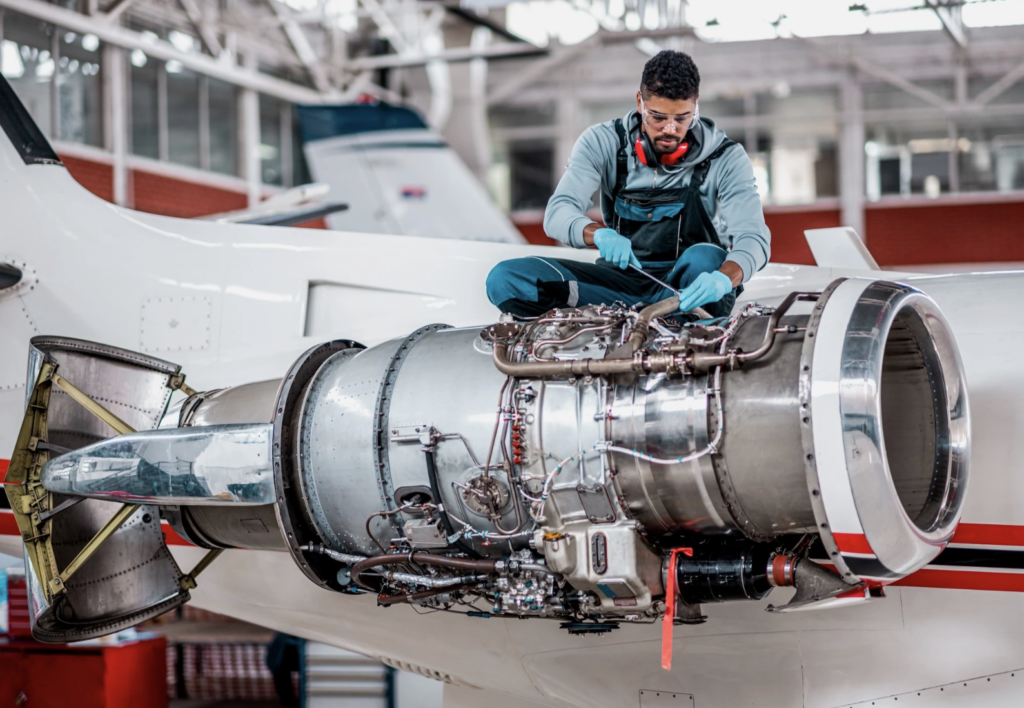In a bustling aircraft repair facility, a young Black mechanic, likely in his twenties, is meticulously working alone on a jet engine mounted to a plane. The photographic image captures him in blue coveralls over a blue shirt, with red ear protectors resting around his neck and safety goggles shielding his eyes. He wears blue latex gloves and wields a tool resembling a slender screwdriver, intently focused on adjusting a pipe within the exposed, intricate machinery of the silver jet engine. The engine’s cover has been removed, revealing a labyrinth of wires, tubes, and pipes, as well as identifiable components such as the thrust reverser and annular combustion chamber. The white fuselage of the aircraft, accented with red and blue bands, provides a backdrop to his precise labor. Overhead, the expansive hangar's high ceiling is supported by an array of metal beams, punctuated by windows that let in natural light. A red stripe of paint runs beneath these windows, framing the scene with an industrial charm. Additional aircraft and parts dot the background, emphasizing the workplace setting.